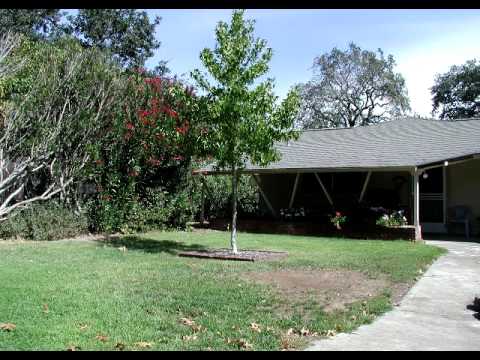The image depicts an outdoor scene in what appears to be a backyard or front yard setting on a sunny day with a blue sky. To the right, there is a driveway leading up to a one-story house with a white front door screen and asphalt shingled roof. The house features a shaded patio supported by pillars, some of which are straight while others form a V shape. The lawn, which spreads across the left side of the image, is green with patches of dry brown areas. Scattered across the lawn are several trees and bushes, including a small sapling and a larger red tree towards the back with either red flowers or fruit. Various plants, some potted, and bushes are positioned along the front and sides of the house. A mix of white and red flowering plants can be seen towards the right side of the image. A notable chair or stool is placed in the right-hand corner near the house.